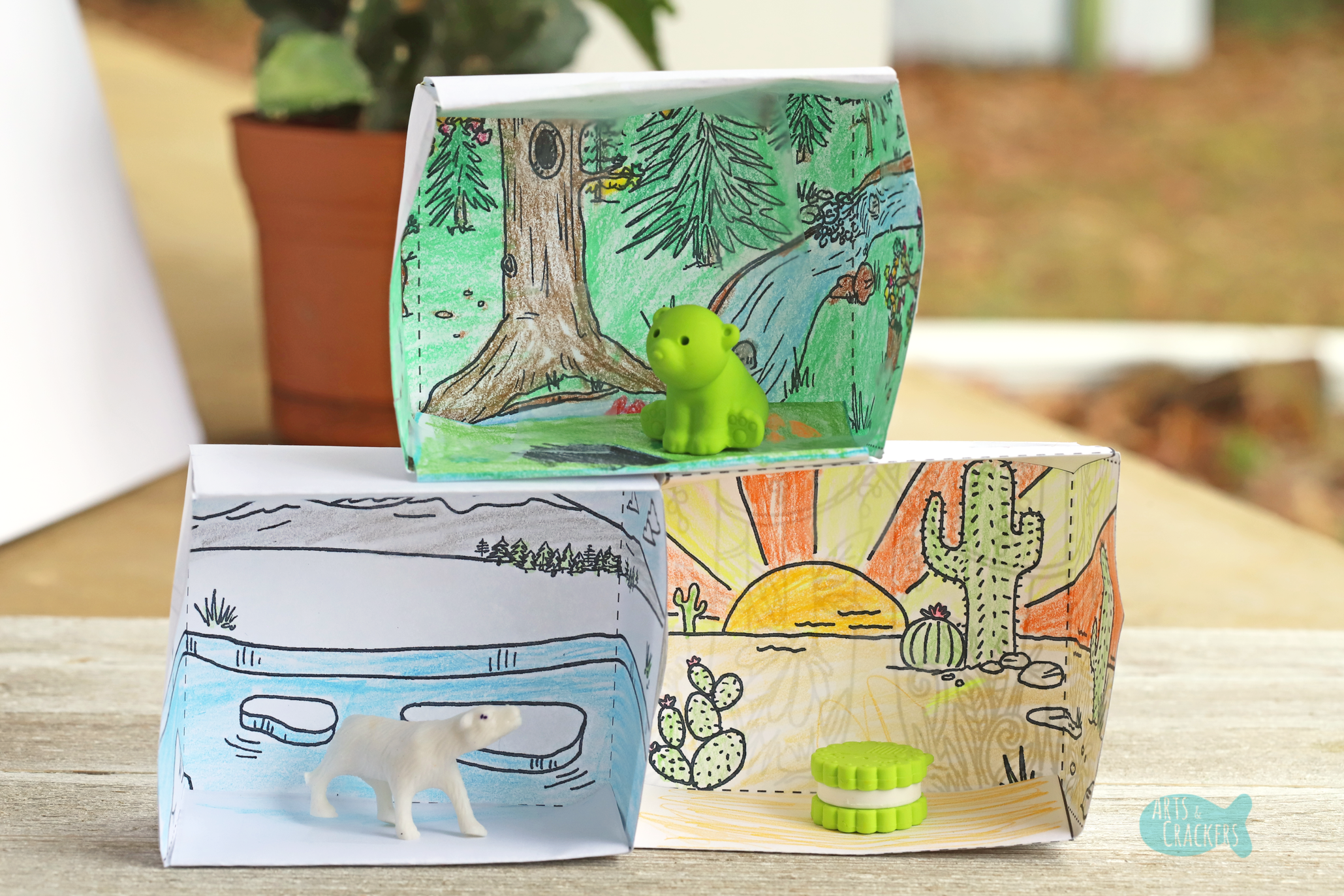This image displays a meticulously crafted children's diorama collection consisting of three nearly square paper boxes, each adorned with vibrant crayon artwork. Two boxes are positioned side by side on a table, with a third box neatly placed on top of them. The leftmost box illustrates a polar landscape, featuring a polar bear figurine amidst floating ice slabs, with snowy mountains and water elements accentuating the background. The right box showcases a desert scene, replete with cacti and a prominent sun with elongated rays, as well as a mysterious green object resembling an oversized Oreo. The top box presents a lush, forest-themed graphic with a river meandering through, a tree with a distinctive hole, and a green koala-like bear at rest. In the backdrop, there's a blurred terracotta pot holding some foliage, adding a touch of real-world greenery to this imaginative display.